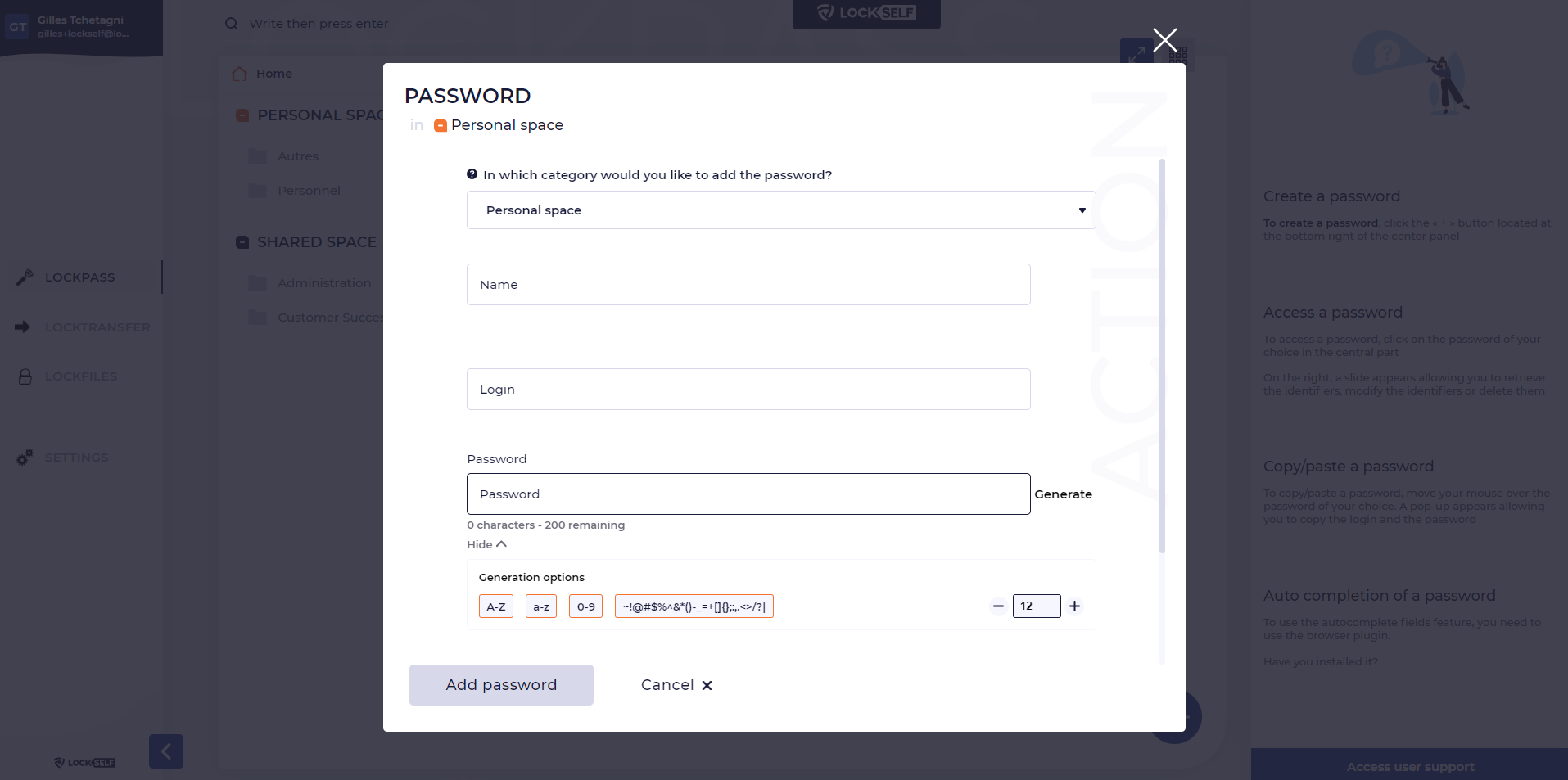In the image, the background features a dark gray shade, partially concealing some scattered papers. In the top-left corner, a black box is faintly visible. Dominating the central area is a large white box crossed with a bold white 'X' and labeled "Password." Adjacent to this is a small orange block bearing the inscription "Personal Space," accompanied by a tiny blue dot. 

Embedded within the white box is a prompt: "In which category would you like to add the password?" Below this, another significant white block is titled "Personal Space," with a downward arrow next to it, suggesting a dropdown menu.

Further down, a large block is labeled "Name," followed by another labeled "Login." Below these fields, the section "Resources" is listed, bordered by black lines on each side and underlined with a blue line that repeats the text "Password." To the right, a "Generate" button is positioned alongside the box.

A counter indicates "200 characters remaining." Nearby, a small word sits next to an up arrow. The section titled "Conversation Options" contains several blue-boxed characters, each outlined in red. 

At the bottom, a blue button reads "Add Password," and a white button labeled "Cancel" is paired with a blue 'X.' Just above these buttons, two blue lines feature a minus sign, the number 12, and a plus sign, likely for incremental adjustments. Finally, a blue scroll line is situated on the right-hand side, with an indistinguishable word beneath it.